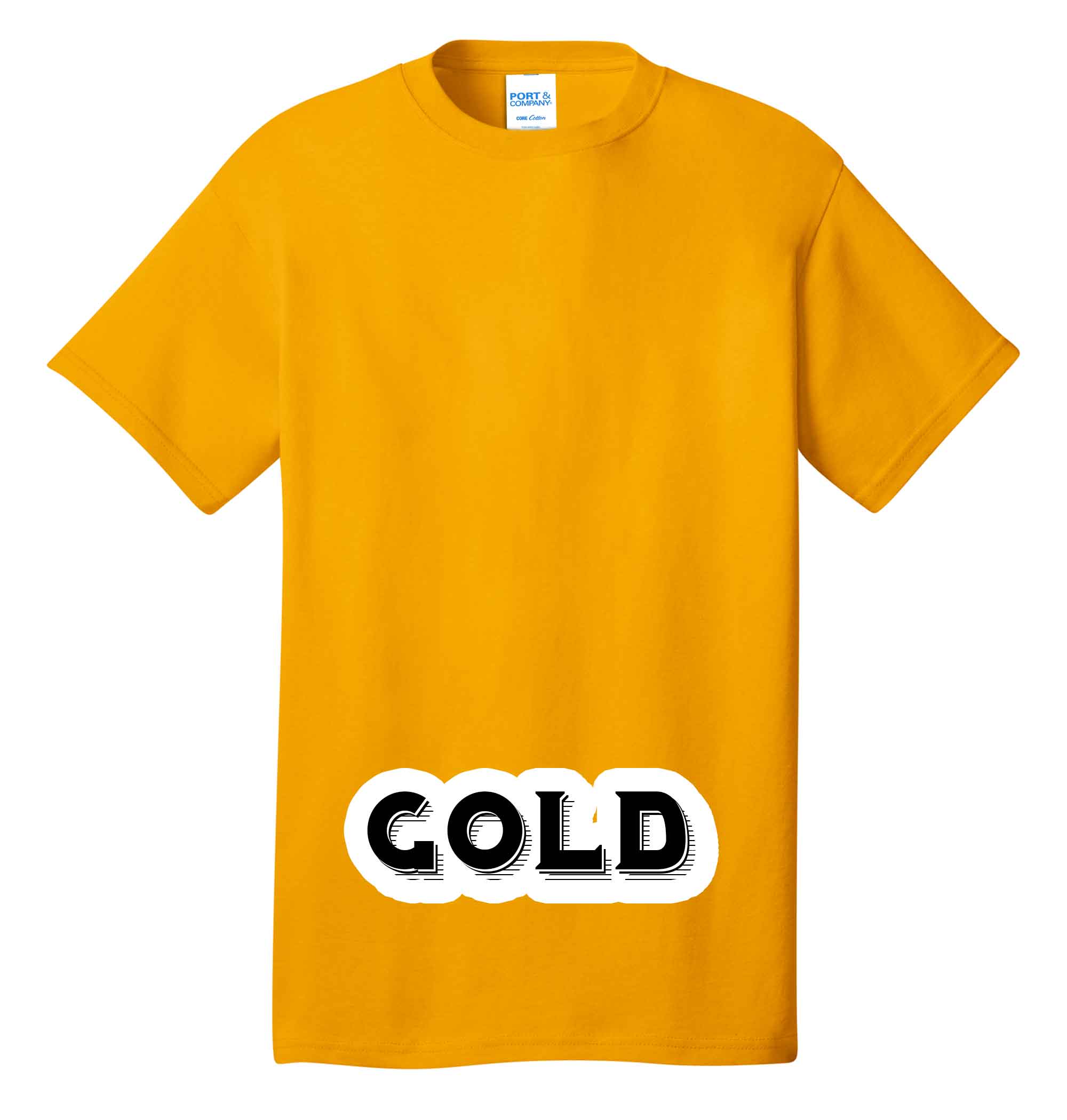This is a vertical photograph of a gold-colored t-shirt with short sleeves and a tight neckline. The shirt appears to be long and features a manufacturer's label inside the neck, which presumably provides product information. Notably, the bottom of the shirt showcases bold black letters that spell "GOLD," outlined in white. This white outline seems to overlay a larger, squished white version of the word "gold" in the background. The backdrop of the image is a plain solid white, giving it the feel of a stock image suitable for a clothing website. There are no additional objects in the image, keeping the focus entirely on the t-shirt. The shirt itself is positioned centrally, emphasizing its design and the text on it.